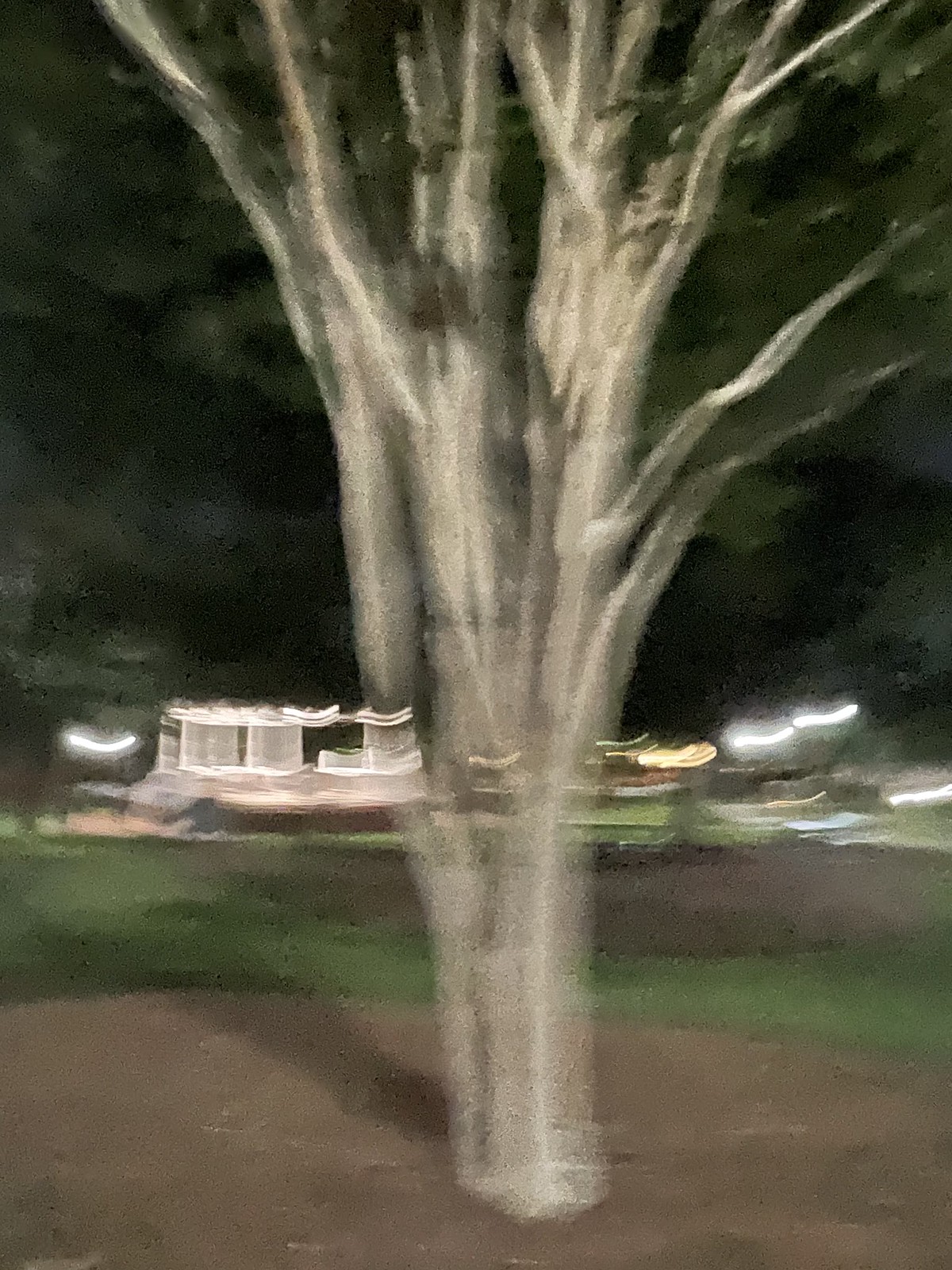The photograph, though blurry and taken at night, centers on a predominantly white, leafless tree emerging from a circular patch of brown dirt in the foreground. The tree's light gray trunk reaches upwards with sparse, vertical branches. Beyond the tree lies a grassy area, and in the distance, a cluster of trees with visible leaves surrounds a brightly lit structure. This structure, possibly a house adorned with white strands of Christmas lights, casts a warm glow, creating reflections and squiggly light patterns that illuminate the scene. The overall image, though dark and indistinct, captures an atmospheric outdoor setting with a mix of natural elements and festive decorations.